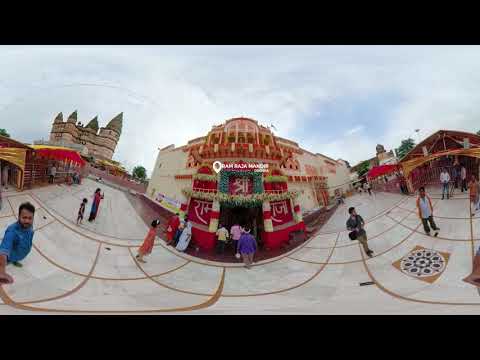The image is a heavily distorted 360-degree panoramic photo of a bustling courtyard area in what appears to be an Asian or Indian market town. Every object in the image is warped with a distinctive U-shaped curvature, where items on the right and left are bent upward, and those in the center curve downward. Near the left edge, a man dressed in blue is holding a selfie stick, indicating he is the one taking the photo. He has black hair and brownish skin. The courtyard itself has a grid-like pattern with squares of gray cement, each outlined with golden trim.

In the center of the image, directly facing the camera, stands a shop-style building characterized by its elaborate red archway adorned with green plants and flowers. To the right of this building is a red tent area, likely part of a marketplace. Further off in the distance to the left, a tall, castle-like building with white sides and four green, pointed tops adds a majestic backdrop to the scene. The sky is a light blue and slightly overcast, adding a soft ambiance to the overall colorful and vibrant setting. People in the courtyard appear to be casually walking around or shopping, enhancing the lively atmosphere of this distorted yet captivating image.